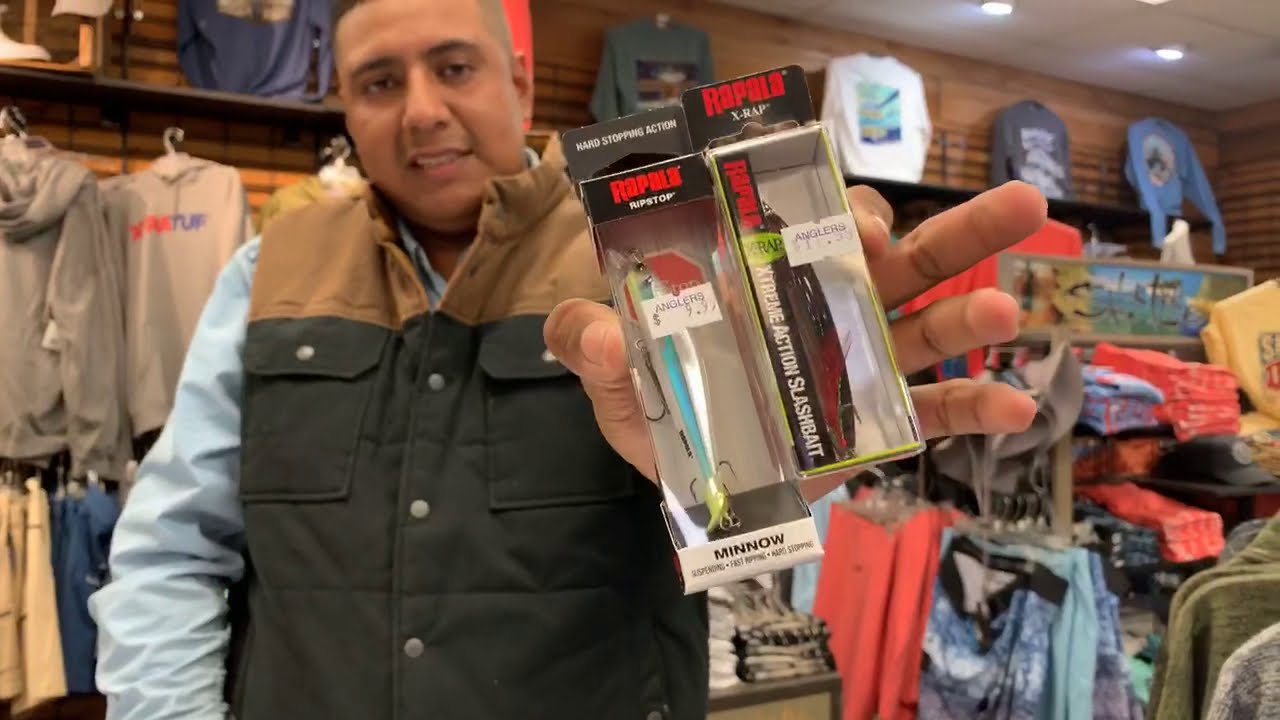The scene captures the interior of a sporting goods store, with a focus on a dark-skinned gentleman positioned in the foreground. The man has dark hair and eyes, and he wears a black vested jacket with beige accents over a blue long-sleeve shirt. He is holding two Rapala fishing lures in his outstretched hand: one labeled as Minnow in black letters on a white background, and the other labeled Extreme Action Slash Bait in white letters. The store's background features rows of clothing items, including hoodies, long-sleeve t-shirts with graphics, shorts, and shirts in various colors such as gray, tan, blue, white, yellow, and red. The back wall is made of wood-paneled horizontal strips, illuminated by recessed lighting. The man appears pleased, possibly promoting the fishing lures. The overall style of the image is photographic representationalism.